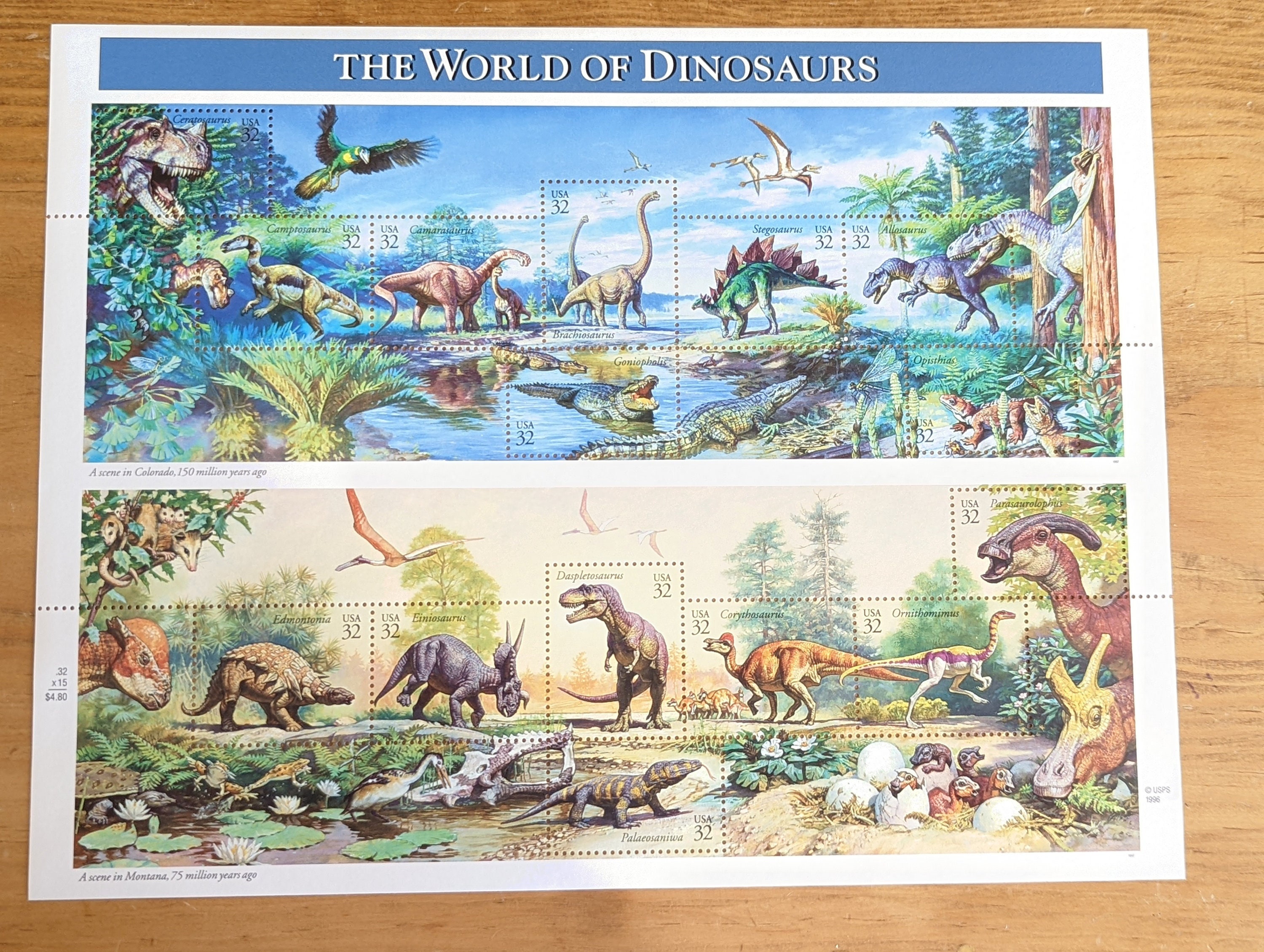The image features a sheet of commemorative postage stamps titled "The World of Dinosaurs," laid out on a wooden table. The sheet is divided into two distinct scenes, each adorned with perforated outlines around various dinosaurs, each marked with "USA 32," indicating their value. 

The top half of the sheet illustrates a rich, watery habitat, possibly a swamp or near a large water body, teeming with diverse dinosaurs like T-Rexes, Brontosaurs, Stegosauruses, and Pterodactyls, all surrounded by trees and various bits of foliage. The intricately detailed scene captures approximately 10 to 20 dinosaurs and birds, each highlighted within the dotted perforations, creating the impression of a vibrant prehistoric ecosystem.

In contrast, the bottom half depicts a drier, scrubby landscape reminiscent of the Serengeti, featuring a large central path and a small pool to the left. This scene also showcases multiple dinosaurs, including a nest of eggs, depicted in perforated sections that emphasize individual creatures. The overall arrangement of the stamp sheet suggests a thoughtful blend of art and functionality, making it suitable for collection, framing, or use as actual postage stamps.